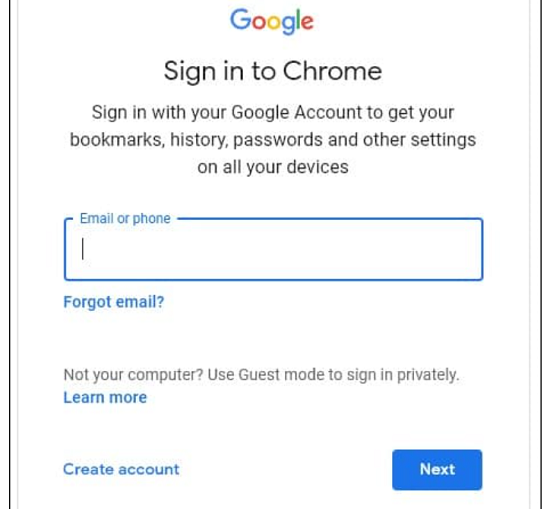The image depicts a partial screenshot of a phone display showing the Google Chrome sign-in page. At the top, the familiar Google logo appears in its classic colors: blue, red, yellow, blue, green, and red. Centered beneath the logo, large, thin, black text reads "Sign into Chrome." Below this, in a smaller font of light black, there's an instruction: "Sign in with your Google account to get your bookmarks, history, passwords, and other settings on all your devices."

A large, blue text box is prominently featured. In the upper left-hand corner of this box, there's a field labeled "Email or phone," with a blinking cursor indicating where the user can input their information. For those who might have forgotten their email, there's a selectable option beneath the input field that says "Forgot email?". 

Further down, there's a notice: "Not your computer? Use Guest mode to sign in privately," followed by a clickable "Learn more" link for additional information. At the bottom of the display, the option "Create account" is visible for users who need to set up a new Google account.

If the information is correctly entered in the email or phone field, users can proceed by clicking the blue "Next" button. The button is clearly marked with the word "Next" in white text, ready to advance the user to the next step in the sign-in process.